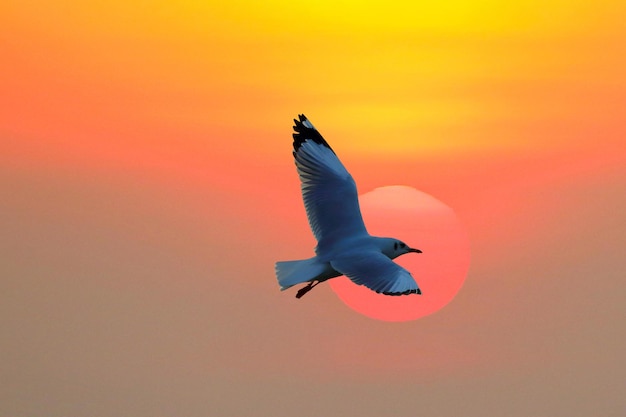A detailed painting captures the moment of a blue seagull flying in front of a vibrant sunset. The bird, positioned centrally in the image, boasts outstretched wings with black feather tips and black accents on the back of its wings. Its long black beak, black eyes, and black spot behind the eyes are distinct. The seagull has patches of lighter white and light blue on the tips of its wings and a lighter tail. The bird's feet, hanging slightly to the left, appear black. The sun behind the bird is a pink circle with a cream-colored top, partially obscured by the bird. The sky transitions from a vibrant yellow at the top to a light pink, eventually turning brown as it descends. This beautiful gradient captures the serene yet striking hues of a sunset, enhancing the overall aesthetic of the nature scene.